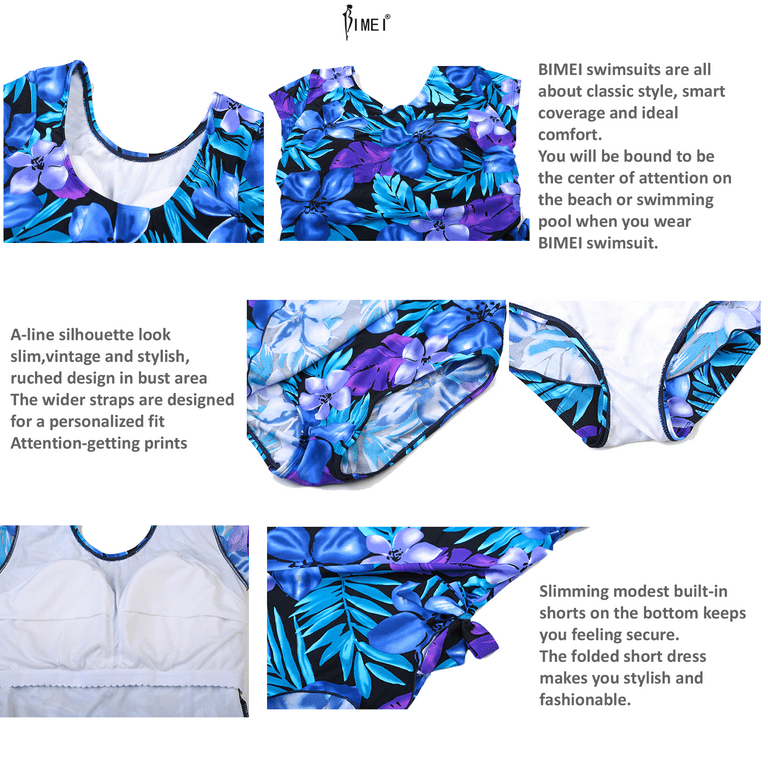This image presents a detailed visual showcase of a B-I-M-E-I swimsuit through a series of up-close photographs arranged in panels. The swimsuit features a striking Hawaiian floral pattern in blue and purple hues against a black background, set on a white base.

At the very top, the brand name "B-I-M-E-I" is prominently displayed in black letters. The top row includes detailed shots of the front and back of the swimsuit, resembling a t-shirt shape, with the accompanying text highlighting that B-I-M-E-I swimsuits offer classic style, smart coverage, and ideal comfort, ensuring you will stand out at the beach or pool.

The center row provides close-ups of the swimsuit bottoms, showcasing the outside and inside views. Text annotations describe the A-line silhouette, which looks slim, vintage, and stylish, along with a ruched design in the bust area. The wider straps are specifically designed for a personalized fit, featuring attention-getting prints.

In the bottom row, the interior of the swimsuit top and a close-up of the side are depicted. The description points out the modest built-in shorts that offer a sense of security, and the folded short dress style adds a touch of fashion and elegance. Overall, the series of images and descriptive text paint a comprehensive picture of the B-I-M-E-I swimsuit's design, style, and unique features.